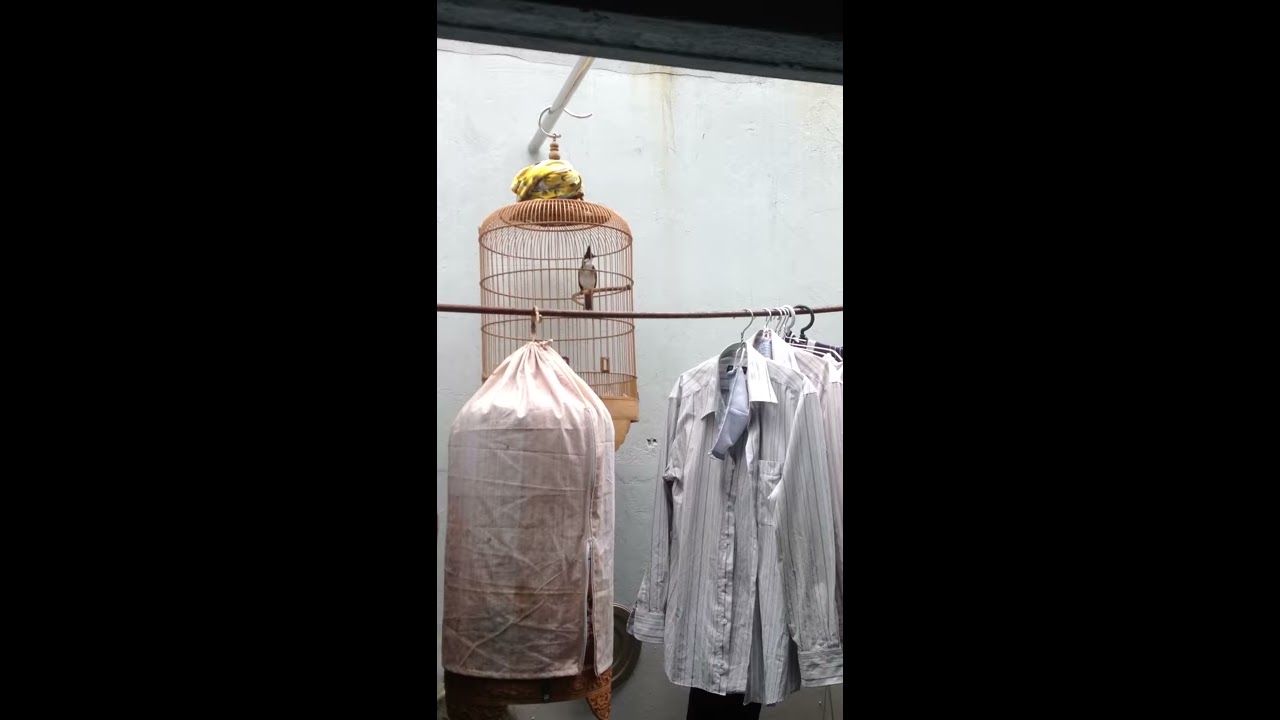The image features numerous birdcages and clothing suspended from wires against a stark white wall marked with signs of rust or mold near the top. Dominating the center top of the frame, a classic, brown metal birdcage dangles from a hook on a pole, housing a white and black bird perched inside, facing forward. In front of this central birdcage, another cage of similar design hangs from a different line, shrouded in a thin, see-through curtain. To the right of these birdcages, a collection of buttoned-up t-shirts hangs from the same line, each white or striped. The most prominent garment among them is a collared, long-sleeved, button-up shirt, accompanied by a face mask on the same hanger.